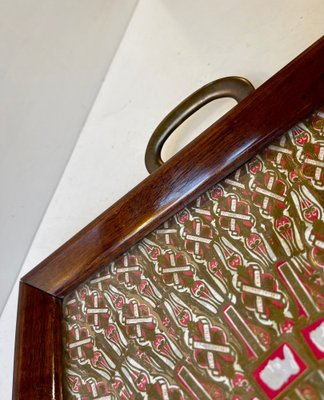This photograph depicts a meticulously crafted wooden drawer or tray situated on a pristine white surface, likely a table or floor, adjacent to a white wall. The drawer features a smooth, polished wood finish, accentuated by a gleaming metal handle positioned at the center right of the image. The interior of the drawer is adorned with intricate golden textures depicting figures with crossed arms or X-shaped designs, arranged in a repeating pattern of golds and whites. Additionally, the bottom right corner of the drawer contains a couple of notable red and white stickers or emblems. The remarkable polish and shine of the wood around the edges indicate that the drawer is well-maintained and appears almost new. The combination of detailed gold designs and the peculiar inclusion of stickers adds a layer of intrigue to this elegantly constructed piece.